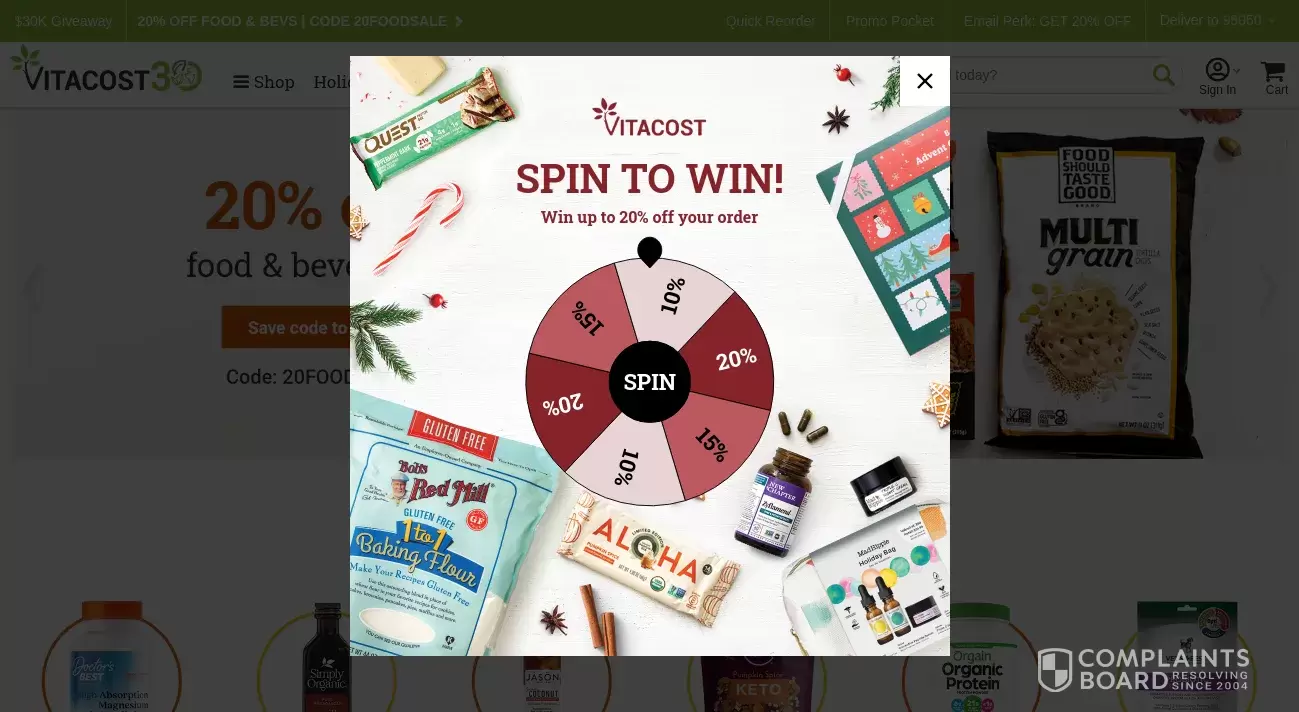This wide-format image appears to be a screenshot from the Vitacost website, a company specializing in mail-order health supplements and organic products. At the top, a green banner prominently announces in white text: "Fast and Free Shipping. 15% Off Supplements, Sports and Diet. Use Code: STRONG." On the right side of the banner, features like "Quick Reorder," "Promo Pocket," "Email Perks—20% Off," and "Deliver to 95101" are displayed.

Below this is a white banner featuring the Vitacost logo alongside navigation tabs labeled "Shop," "Heart Health," "Tips and Recipes," and "Deals." A search bar prompts with the query: "How can we help you today?" 

Dominating the center of the page is a sizable advertisement for "15% Off Supplements, Sports, and Diet" with a call-to-action to use the discount code "STRONG." An image showcases various open containers of vitamins and a bag of Quest Mini Peanut Butter Cups.

Further down, a section titled "Deals You'll Love" presents six featured products, each encircled by alternating blue and teal borders. Notable items include "Pacific Organic Cream of Mushroom Soup" and a "Magnesium Complex Supplement."

This screenshot offers a comprehensive glance at Vitacost's offerings, user interface features, and ongoing promotional deals, encapsulating its focus on health-related products and consumer convenience.